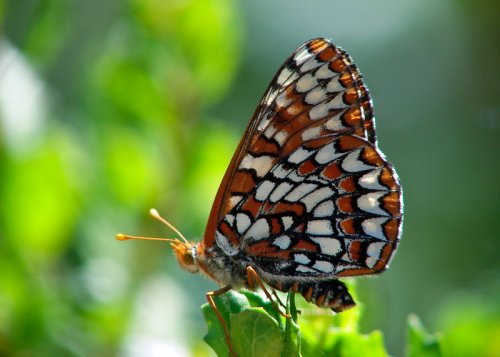This captivating image showcases a stunning butterfly perched on a single, broad-shaped green leaf. The butterfly's intricate wings are held upright, displaying their vibrant underside adorned with an array of colors—black, gold, rust, and white. Its delicate wings, with an orange base and white markings outlined in black, nearly reach the top edge of the frame. The butterfly's golden head, with matching gold antennae tipped in yellow, and brown eyes, add to its enchanting appearance. The body exhibits a striking contrast: black on top, with a white, black, and gold-patterned underbelly. Surrounding the butterfly, the out-of-focus background of light and dark green leaves accentuates the sharp, detailed beauty of its subject.